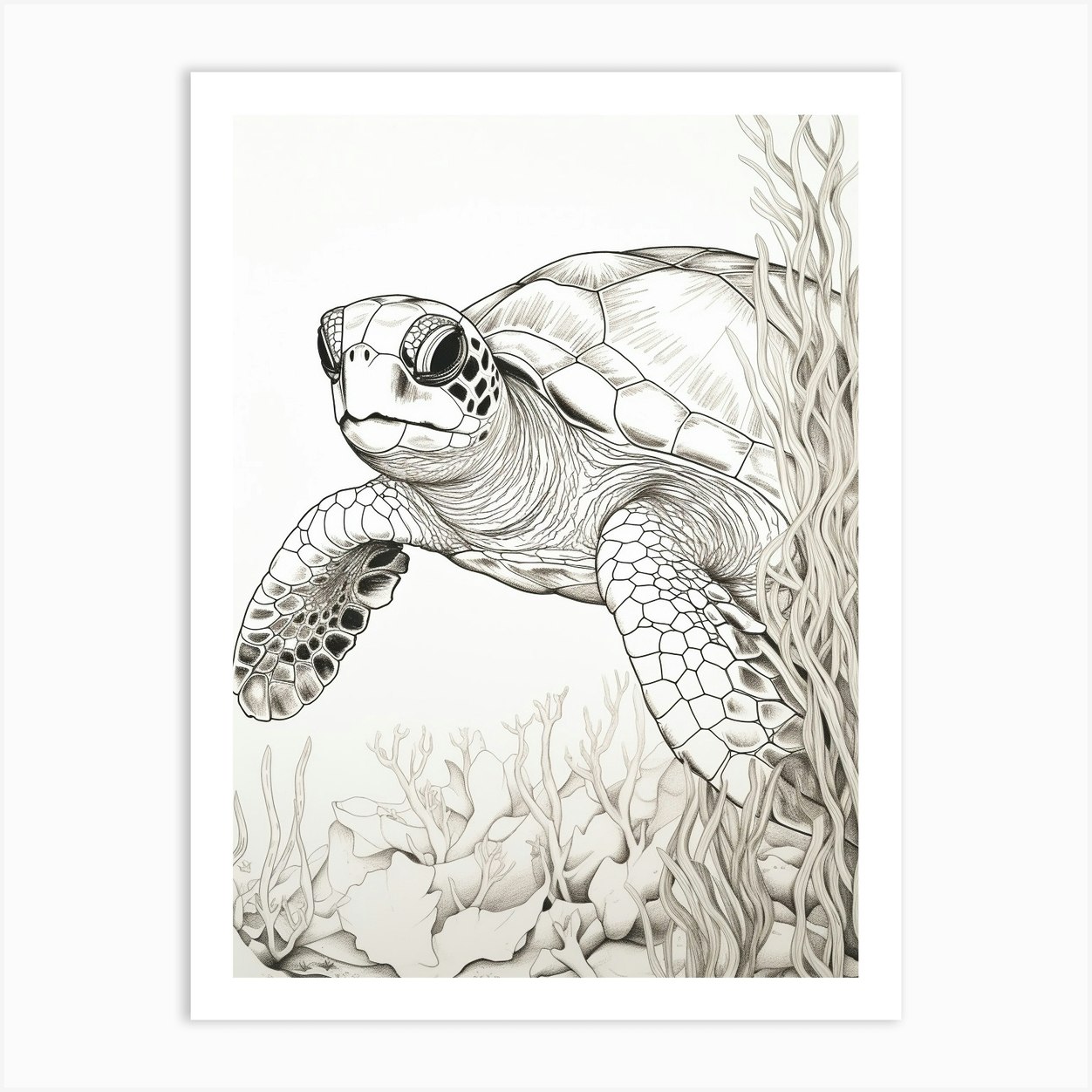This image portrays a highly detailed black-and-white drawing of a sea turtle, expertly shaded to create depth and texture. The sea turtle, the main focus of the drawing, is depicted swimming gracefully through its underwater environment. Its large, dark eyes and pronounced features capture attention. The turtle’s meticulously drawn scales on its fins and shell highlight the artist's skill in shading and detail. Below the turtle, intricate drawings of coral and seaweed add richness to the scene. These underwater plants, especially the tall seaweed on the right that extends from the bottom to the top of the picture, enhance the sense of the turtle navigating through the ocean. The simple, plain white background ensures that the turtle and its surroundings are the primary focus, making this an elegant and captivating piece of art.